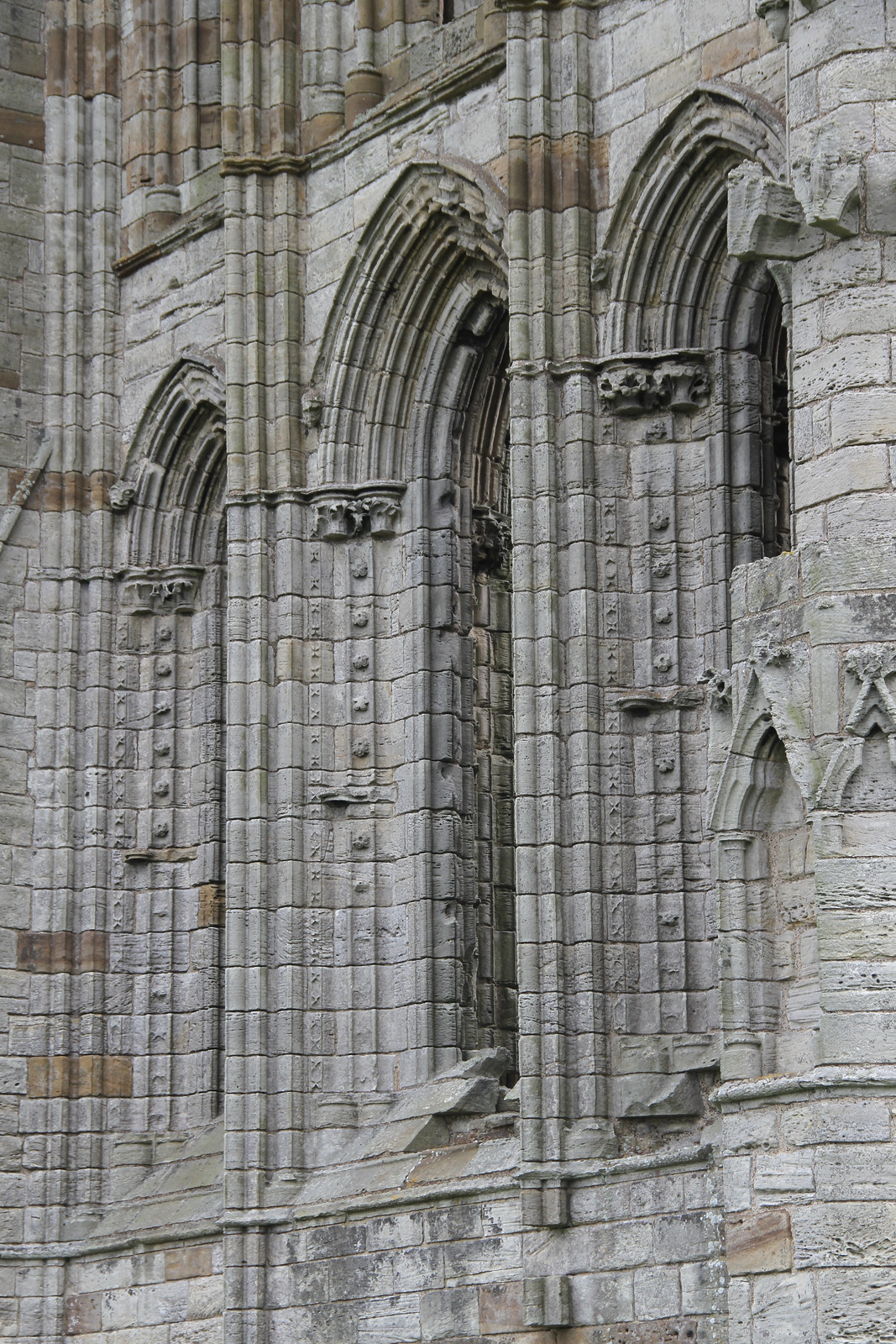This is a detailed photograph of a section of a cathedral’s facade captured in portrait orientation at an angle, showcasing its gothic architectural style. The image highlights three prominent arches that likely once housed windows. These arches are framed by sturdy, ornate columns made of primarily gray stone, with some brown stone details at the top. Vertical architectural edgings enhance the gothic style, contributing to the overall intricate design. The facade features large stone bricks with some squares adorned with embellishments. Notably, on the right side of the image, perched on the columns, are some gargoyles. The top and bottom portions of the image reveal a combination of gray and brown stones, with some engraved stones suggesting elements like vases.